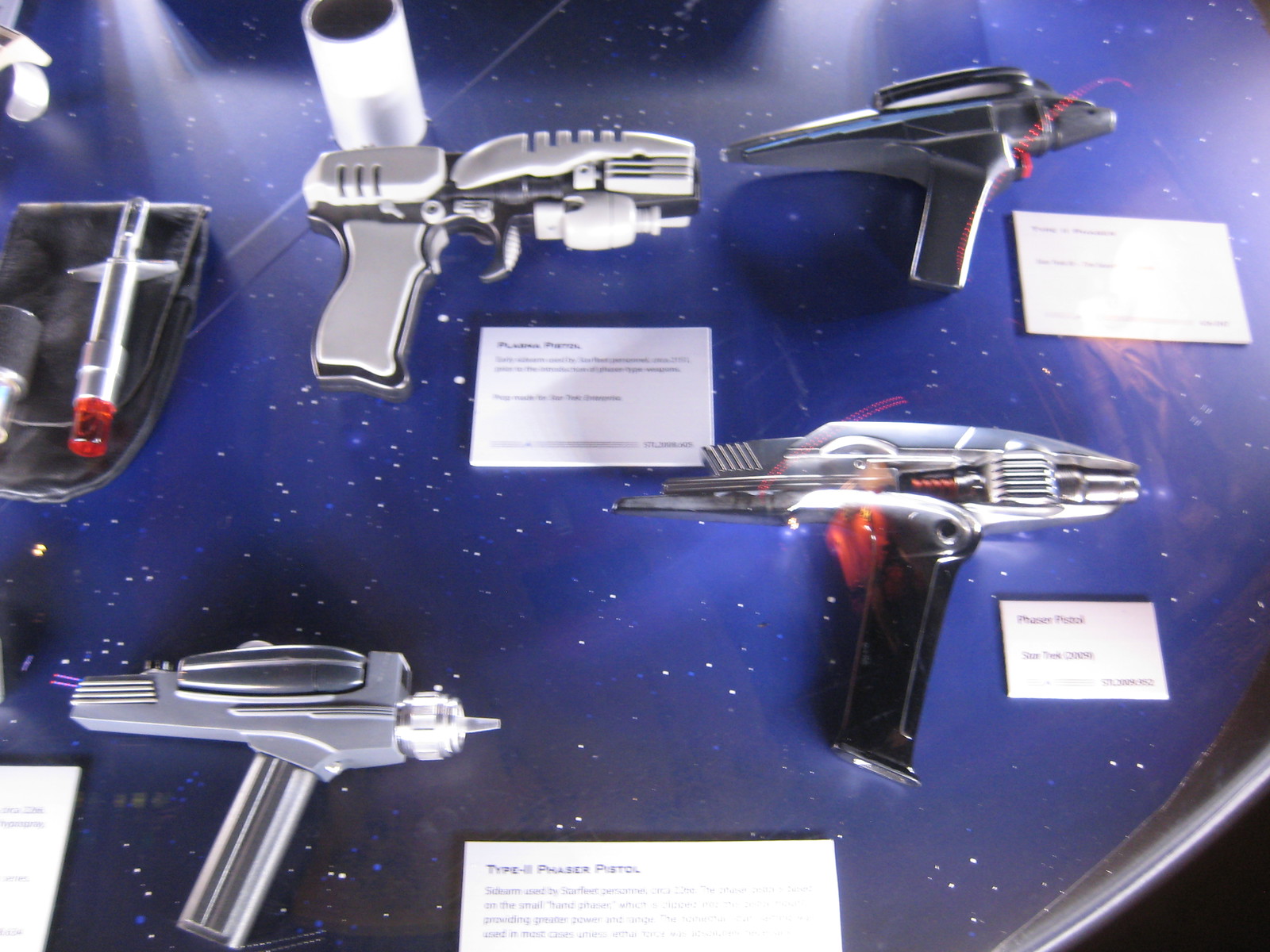The photograph, taken indoors, captures a rectangular display of sci-fi prop guns arranged on a tabletop. The background of the display case is a deep royal blue, adorned with small white, blue, and purple flecks to emulate a galaxy full of stars and distant planets. The display features a total of five gun-shaped props, evocative of futuristic weapons from sci-fi shows like Star Trek or Battlestar Galactica. On the far right, a noteworthy label reads "phaser pistol Star Trek," while another card identifies a "type 3 phaser pistol." Each prop gun has an associated white card with labels, some too small to decipher. Among the various props are a distinctive silver item resembling a hypodermic needle, a silver revolver-like gun, and another with a black handle and silver top. These detailed sci-fi weapons are meticulously laid out, enhancing the overall cosmic theme of the display.